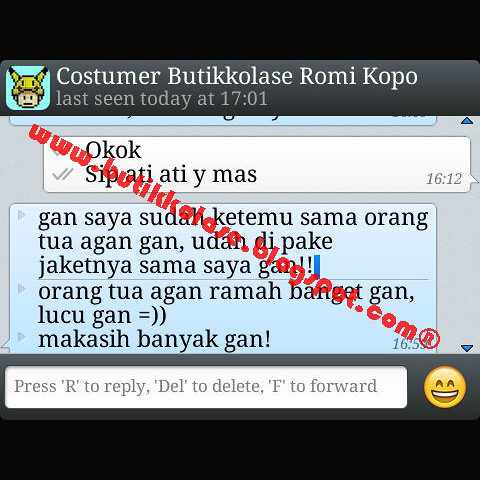This square image showcases a digital chat interface, featuring distinct color elements and structured sections. Dominating the top and bottom edges are thick black horizontal bars. Just beneath the top bar, a dark gray rectangle with rounded corners spans across, highlighting a square icon with rounded corners on its left side. This icon displays a face donning a yellow hat with ears, set against a blue background. To the right of the icon, white font text reads "Customer Butikolase Romi Kopo," accompanied by a gray text below indicating "last seen today at 1701."

The main content area of the chat has a gray background. At the top, a white chat bubble contains the text "okay, okay, sip, adi, adi, imas." This is followed by a blue chat bubble stating "gansai, asuda, kete, musama, orang," and a red chat bubble below that reading "ketsuwa, agangan, udantipake, ketsunayasamasayagan." 

Additionally, elements in the chat interface include a red website address running across the middle, accompanied by a yellow smiley face at the bottom right. Features such as reply (R), delete (needle icon), and forward (F) options are possibly available, inferred from the structure. The color scheme involves light blue, black, yellow, red, and white, contributing to a computer-generated or chat group design where users interact by responding to the group or specific topics.